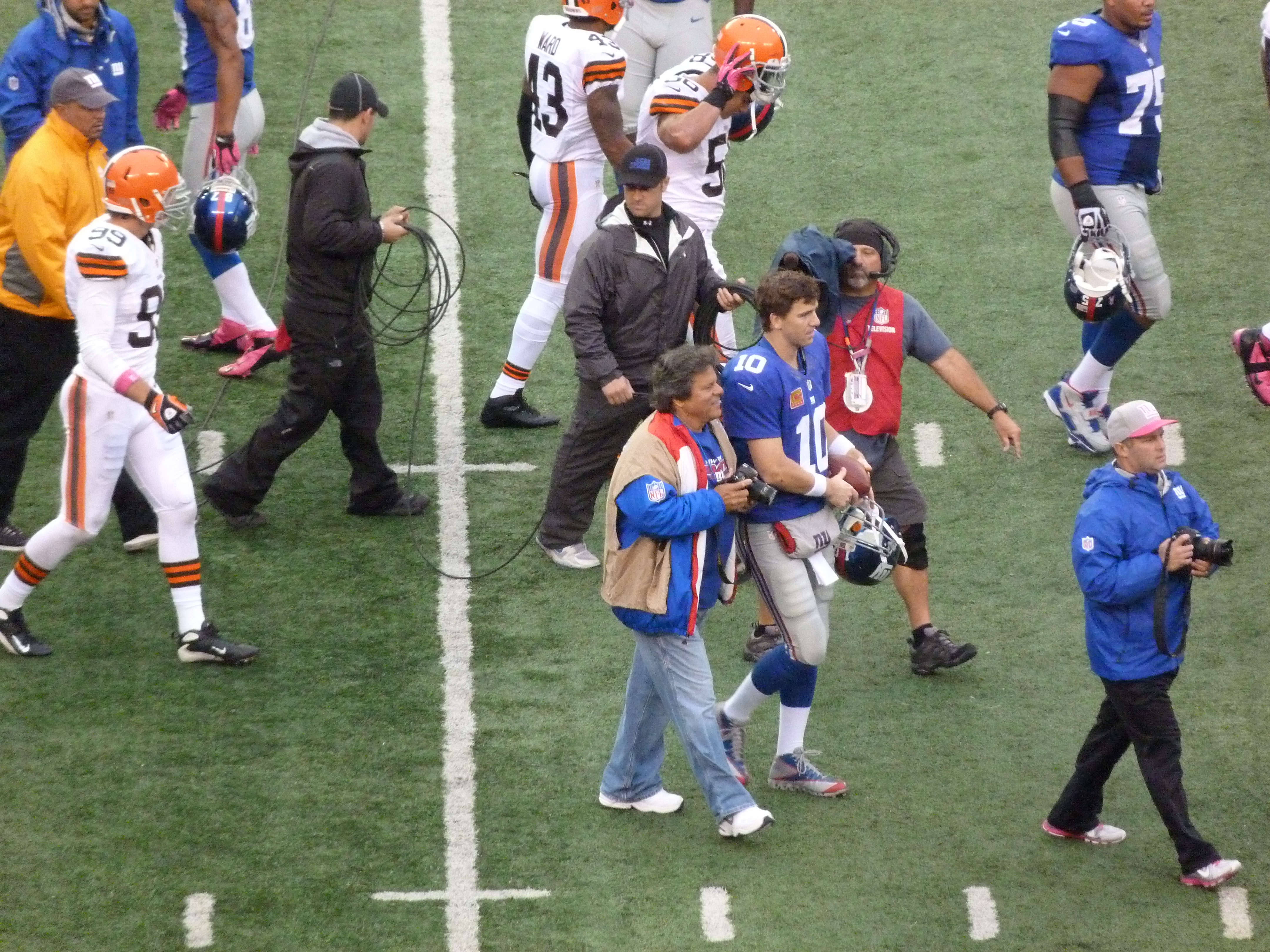The image captures a post-game scene on a football field. At the center is a player dressed in a blue jersey and gray pants, cradling his helmet, and being led off the field by two men—one wearing a red vest, large camera, headset, and mic, while the other is in a blue jacket with a beige vest and jeans, smiling. Surrounding them, several other players in blue jerseys and gray pants mix with at least four players in white uniforms with orange helmets, indicating two different teams. Additional figures include photographers and crew members in black attire, some carrying wires or holding cameras. The background features a green field with white lines and scattered groups of people in motion, suggesting the game has recently concluded.